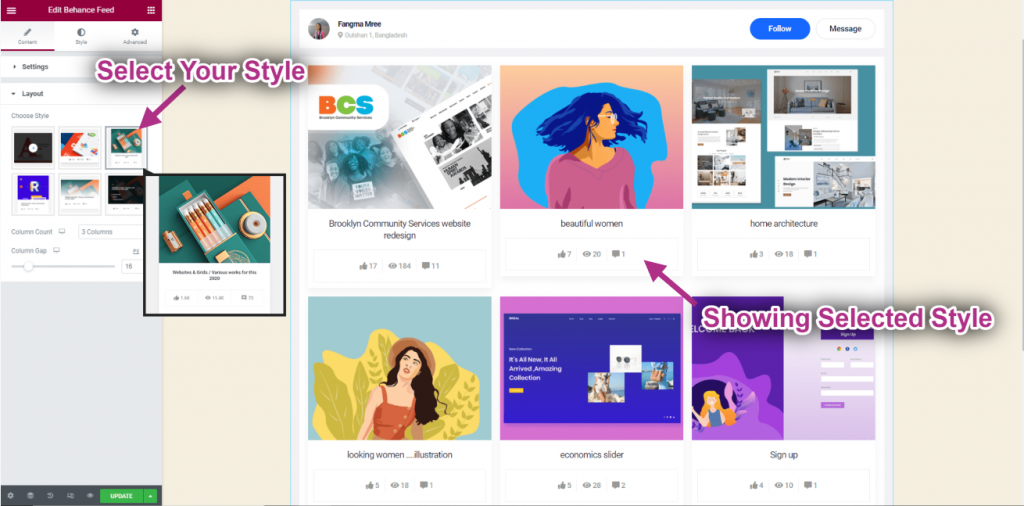This is a screenshot of the backend of a website editor interface. The layout features a sidebar on the left side of the screen and a prominent red bar at the top, displaying the title "Edit Behance Feed." Below this title, there are three tabs each accompanied by icons and text; the first tab is highlighted with an underline in red. 

In the sidebar below the tabs, there are options including a "Settings" button and a "Layout" button. The "Layout" button is expanded, revealing six thumbnail previews of different styles. The third thumbnail in the top row is enlarged, indicating it is the currently selected style. An arrow points to this thumbnail with the instruction "Select Your Style."

On the right side of the screen, a preview of a portfolio website is displayed. This preview includes a name and profile photo on the left, with two buttons labeled "Follow" and "Message," the latter being a blue button. Below this header, the website preview showcases two rows of images, arranged three images per row, providing a glimpse of the portfolio's visual content.